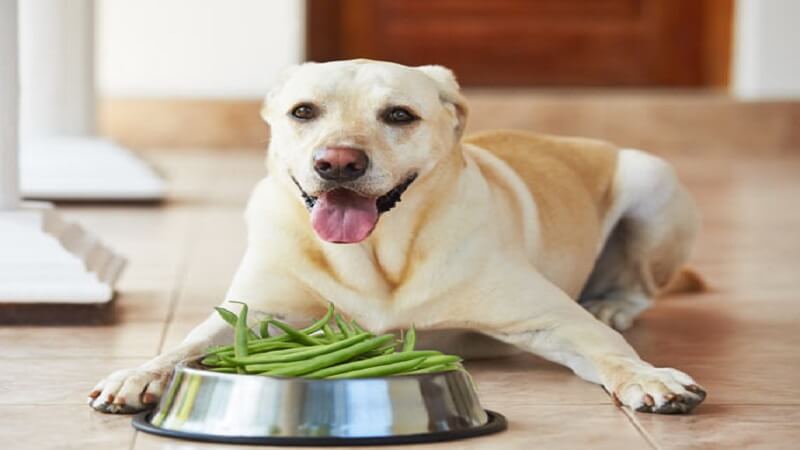A cheerful, light tan dog with a pink and black nose and dark eyes is sitting on a blonde tile floor, staring into the camera with its tongue hanging out. Its front paws are splayed on either side of a silver bowl with a black non-slip rim, which is filled with raw, full-size green beans. The dog’s ears are laid back and it appears content, an expression that seems unusual given the contents of the bowl. The background is blurred, showing the bottom of a wooden door and two white furniture legs to the left, adding depth to the image. The dog's body posture includes its back legs squatting while its stomach rests against the floor.